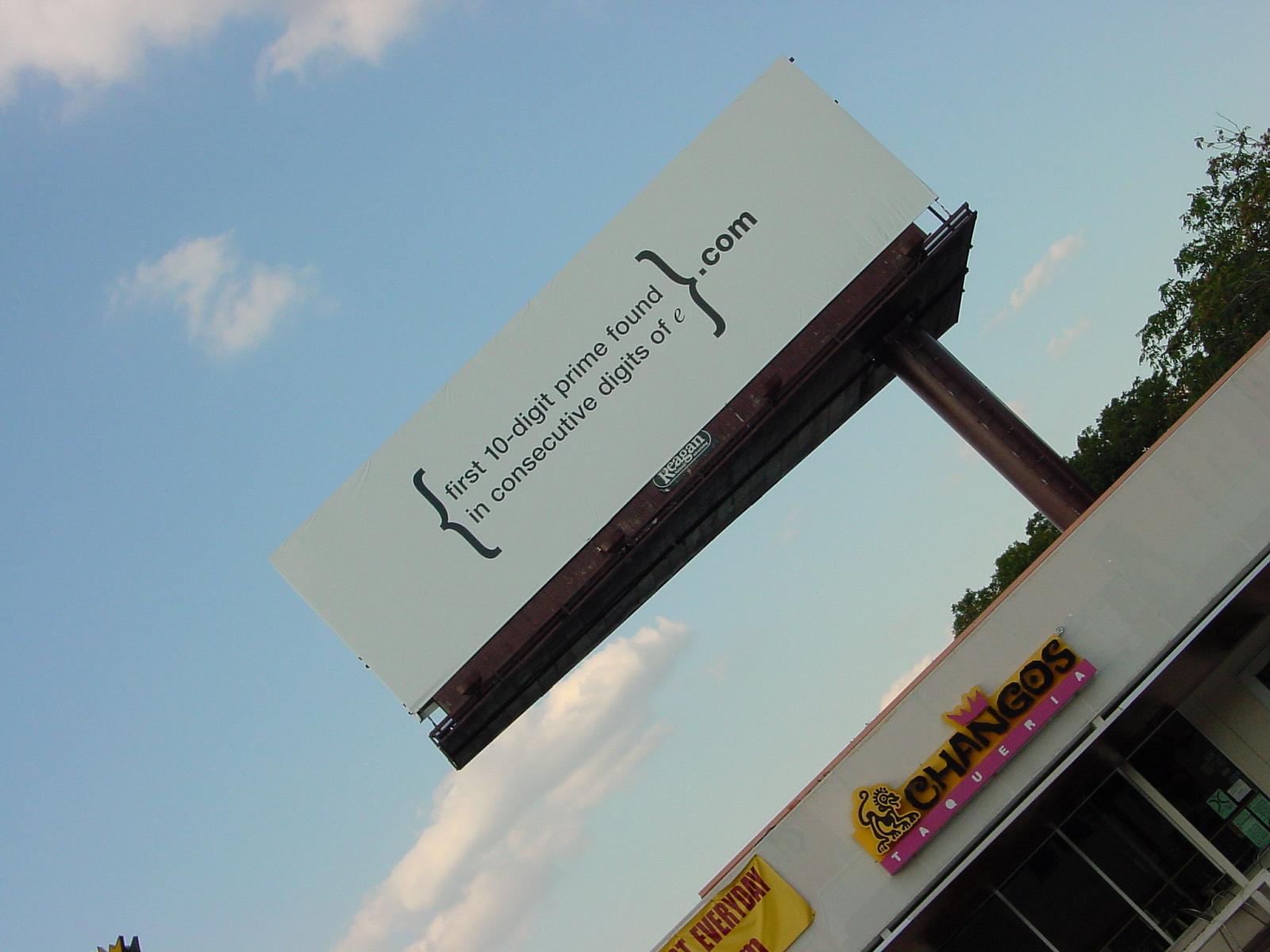This photograph captures an intriguing urban scene featuring a prominently positioned billboard. The billboard is angled at approximately 45 degrees, rising from the left-hand side, and it showcases a thought-provoking message: "First 10-digit prime found in consecutive digits of e.com." Below the billboard, in the foreground, stands Chango's Taqueria, a vibrant restaurant that adds a splash of color to the scene. The taqueria's logo is depicted in a lively black, pink, and yellow color scheme and incorporates a playful black monkey graphic. Adjacent to Chango's Taqueria, on the left, there is a hanging sign which displays the word "every day." The composition of the image, with the juxtaposition of mathematical intrigue and culinary charm, creates a striking and memorable urban tableau.